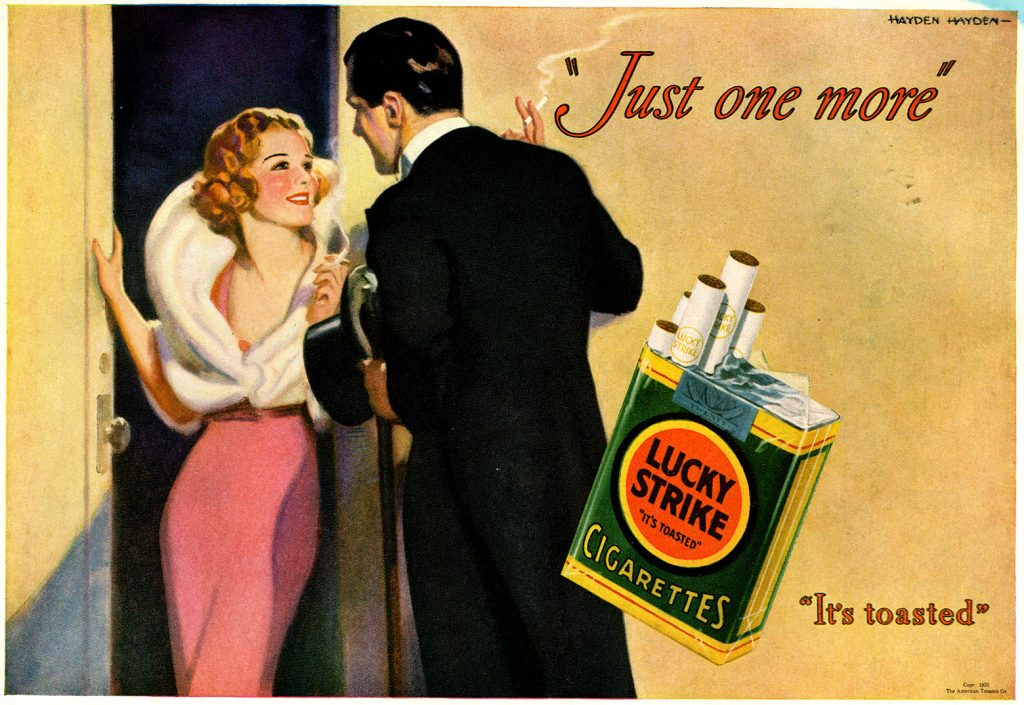This vintage Lucky Strike Cigarettes advertisement, likely from the 1920s or 1930s, features a hand-drawn illustration on a tan background. Dominating the center is a detailed image of a cigarette pack with a couple of cigarettes poking out at the top. The prominent text on the right side of the ad is written in a stylized red font and reads "Just one more" at the top and "It's toasted" in smaller font at the bottom. 

To the left, a man in a black tuxedo, complete with a top hat and cane, stands with his back to the viewer, holding a cigarette in his right hand. Adjacent to him, a woman dressed in a tight-fitting pink dress and a fur wrap leans against a door frame, her hand resting on the door. She has pink blush on her cheeks and also smokes a cigarette. The pair gaze longingly at each other while cigarette smoke drifts between them, capturing the essence of allure and sophistication characteristic of the era's advertising style.